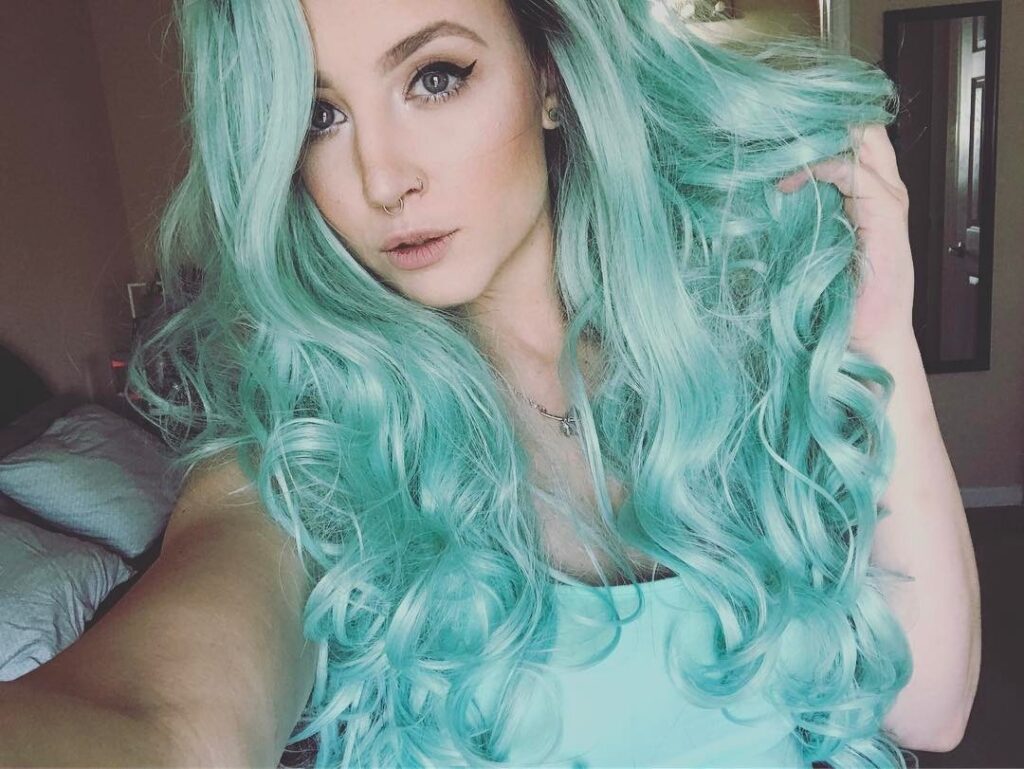The photograph captures a young woman taking a selfie in her bedroom. Her striking blue-green, shiny hair flows down to her mid-torso and is likely newly dyed, as she appears eager to showcase it. Her makeup is meticulously done, with a lot of eyelash eyeliner, carefully shaped eyebrows, and potentially blue-green contacts that match her vibrant hair. She has two nose rings and an earring, and she wears a small metal necklace around her neck. Dressed in a sleeveless white tank top that complements her hair color, she poses with one hand holding her hair up to reveal her ear and the other hand extended out to take the selfie. Behind her, the room decor includes a bed with two pillows, a wall mirror, and a door that presumably leads to a bathroom, illuminated by a light. The walls of the room are tan, and a few other elements like a lamp and a clock can also be seen in the background.